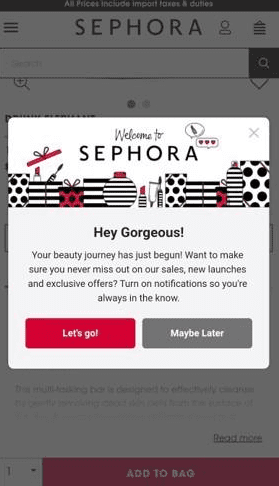In the background, a grayed-out area draws minimal attention, creating a subdued atmosphere. At the top, a sleek, elongated black bar features the word "SEPHORA" in bold, uppercase letters. Directly beneath SEPHORA, a search box awaits user input.

Centrally positioned and commanding attention, a vibrant square prominently displays a welcoming message: "Welcome to Sephora." Below this greeting stands a striking black and white striped gift box, adorned with a black bow and a red top. The box reveals an array of beauty products: a tube of mascara, a vibrant tube of lipstick, and a red and black polka dot box. Further inside the box, additional items in the recurring theme of black, white, and red can be seen, including another tube of lipstick encased in a chic black and white container.

Below this visual feast, the text "Hey Gorgeous!" exclaims in lively black font, inviting the viewer: "Your beauty journey has just begun. Want to make sure you never miss out on our sales, new launches, and exclusive offers? Turn on notifications so you're always in the know." Two clickable options are presented near the bottom: a bold red box with white text urging "Let's Go," and a gray box with a more subdued "Maybe Later" option written in white.